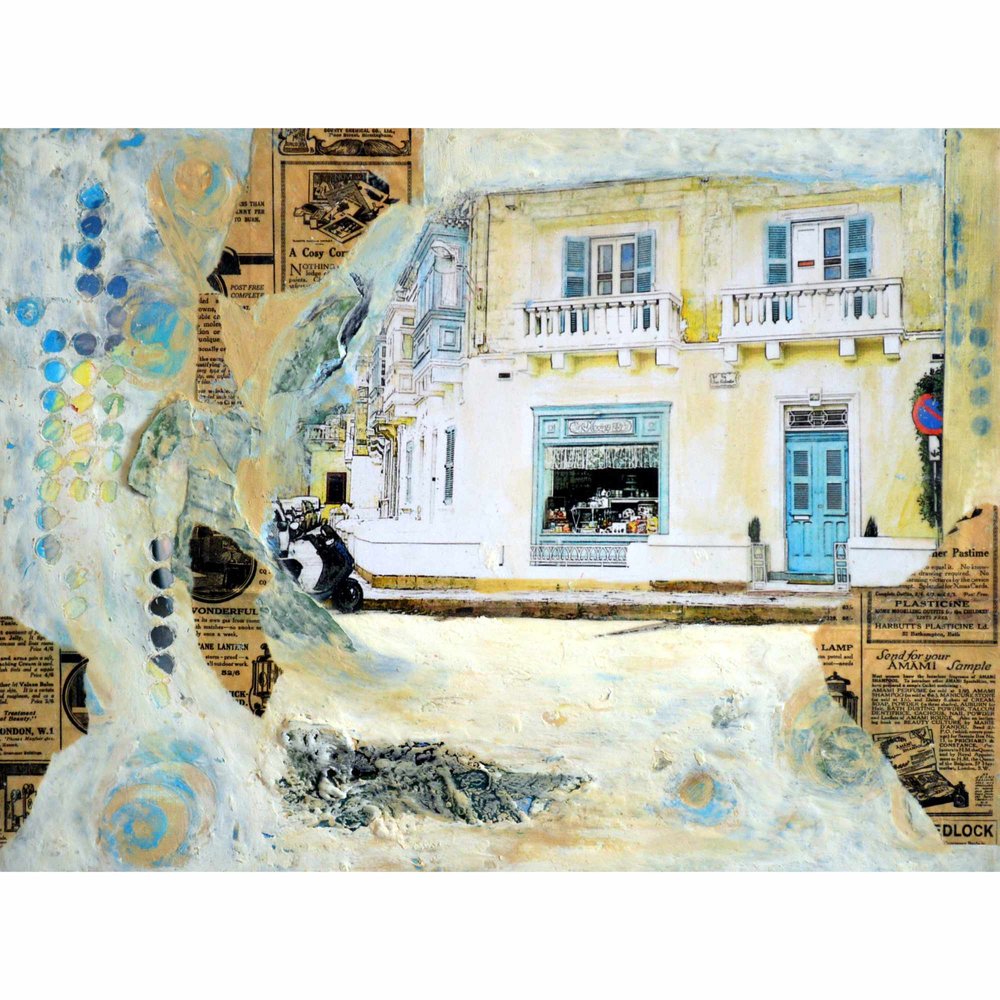The artwork depicts a mixed-media piece featuring a horizontal canvas that combines elements of painting and collage. Dominating the upper right section is a detailed rendering of an old-style European business. This yellow building has distinctive architectural features, including blue double doors on the ground floor and two upper floor balconies with white railings and blue shuttered windows. To the left of the doors, there's a shop window displaying what appear to be bakery goods, though the details are somewhat distant and unclear. The scene also includes a narrow stretch of sidewalk.

On the left side of the canvas, a visually striking area showcases a mix of white, blue, and yellow dots against a backdrop. The background of the entire piece is layered with aged newspaper clippings, characterized by their orange and yellow hues and black print, placed sporadically on the lower right and left sections. These clippings feature old advertisements, adding to the nostalgic and textured feel of the artwork. The lower portion of the canvas exhibits splatters and swatches of paint, lending an abstract quality to the composition, contrasting with the structured depiction of the townscape.